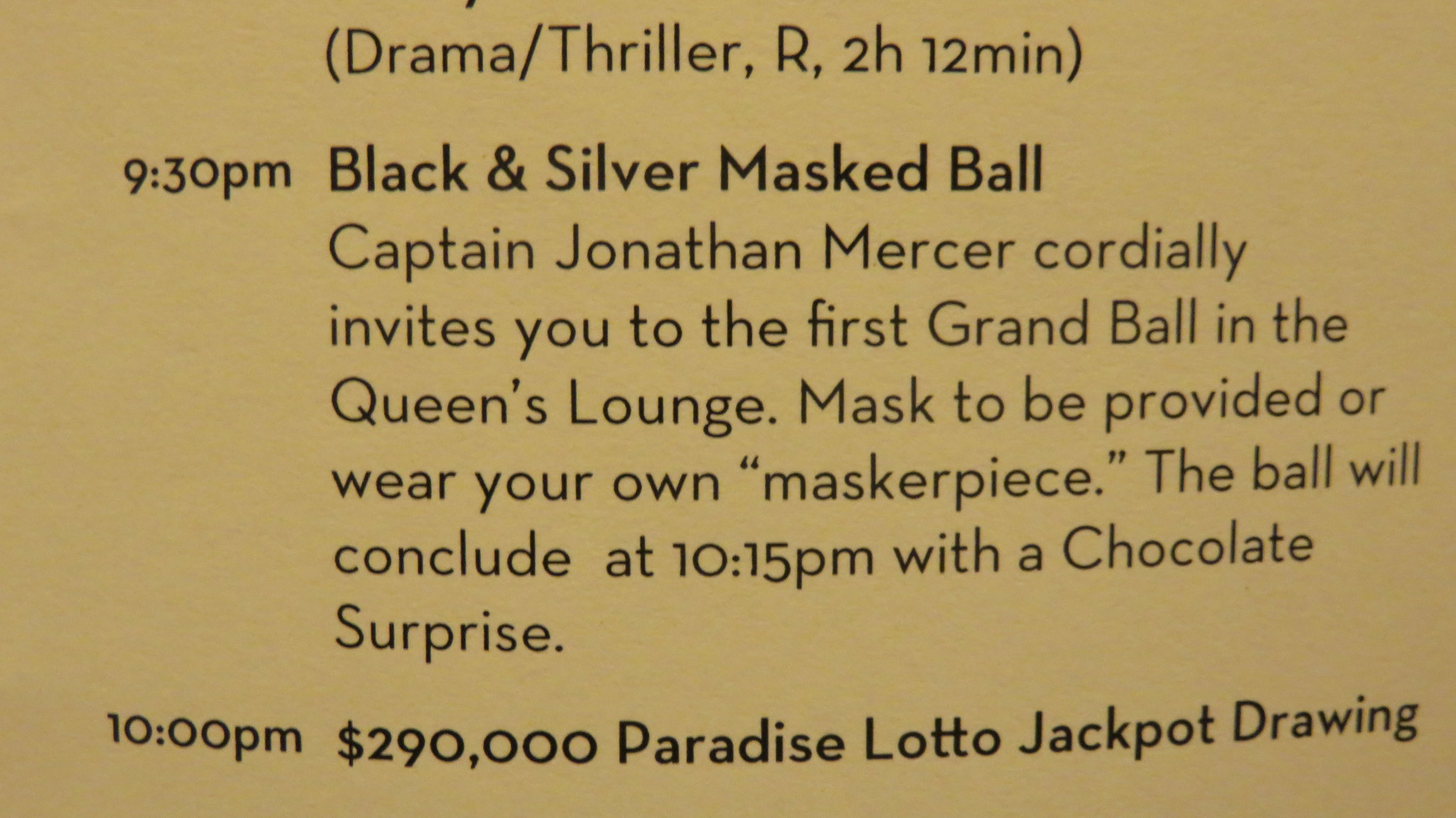This rectangular image, reminiscent of the shape of a high-definition TV, displays text on a yellow background. The black sans serif font is organized clearly, making the information easy to follow. At the top center, it reads "(Drama/Thriller, R, Two Hours Twelve Minutes)." Below this, in bold, it announces "9:30 PM Black and Silver Masked Ball." This event is further detailed in a paragraph that states, "Captain Jonathan Mercer cordially invites you to the first grand ball in the Queen's Lounge. Mask to be provided or wear your own masterpiece. The ball will conclude at 10:15 PM with a chocolate surprise." Following this, another bolded line reads "10:00 PM $290,000 Paradise Lotto Jackpot Drawing."